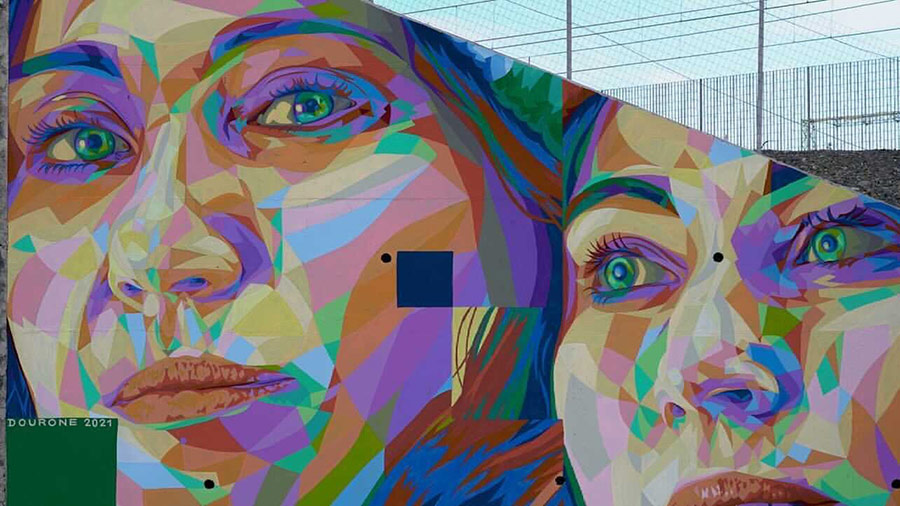The mural depicted in the image is painted on a wall angled higher on the left and lower on the right, bordered by a wire-framed fence and a gravelly hill in the background. The composition features close-up portraits of two women’s faces, rendered through an array of geometric shapes in a cohesive pastel color palette that includes shades of light blue, pink, orange, light yellow, green, and purple. These shapes cut across the faces, forming a detailed yet abstract representation akin to vector art. Notably, a green square in the bottom left corner holds the artist's signature, “Duron 2021,” written in white. Highlighting the vibrancy and intricate style, the faces exhibit pink lips with lighter pink shading, and the colorful geometric shapes accentuate their eyes and cheeks, adding depth and character to the mural.